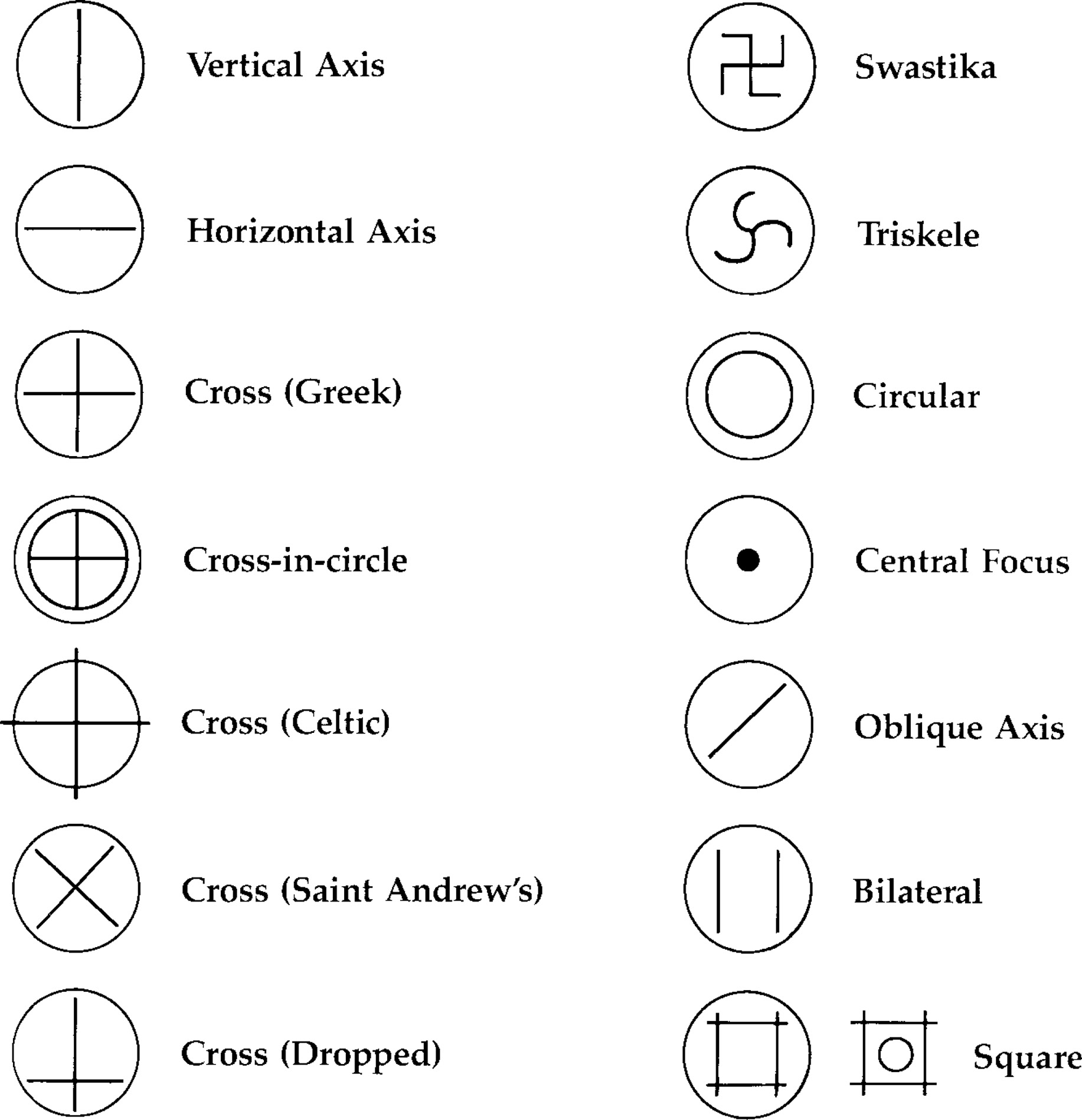The illustration is a meticulously detailed chart featuring a variety of symbols, each accompanied by descriptive text. It is composed of black line drawings on a white background, with most symbols enclosed within circles. The chart is organized into two main columns, each containing a vertical sequence of symbols. The left column begins with a circle intersected vertically, labeled "Vertical Axis," followed by a horizontally intersected circle labeled "Horizontal Axis." Moving down, the symbols progress to a cross, then a Greek cross, followed by a cross encircled, a Celtic cross, a St. Andrew's cross, and finally, a dropped cross. The right column starts with a swastika inside a circle, followed by a triskelion. Further down it features symbols labeled "Circular," "Central Focus," "Oblique Axis," and "Bilateral," with the bilateral symbol depicting two opposite lines within a circle. At the bottom right, the sequence concludes with a square symbol, containing a circle within a larger square formation, uniquely not enclosed by a circle.